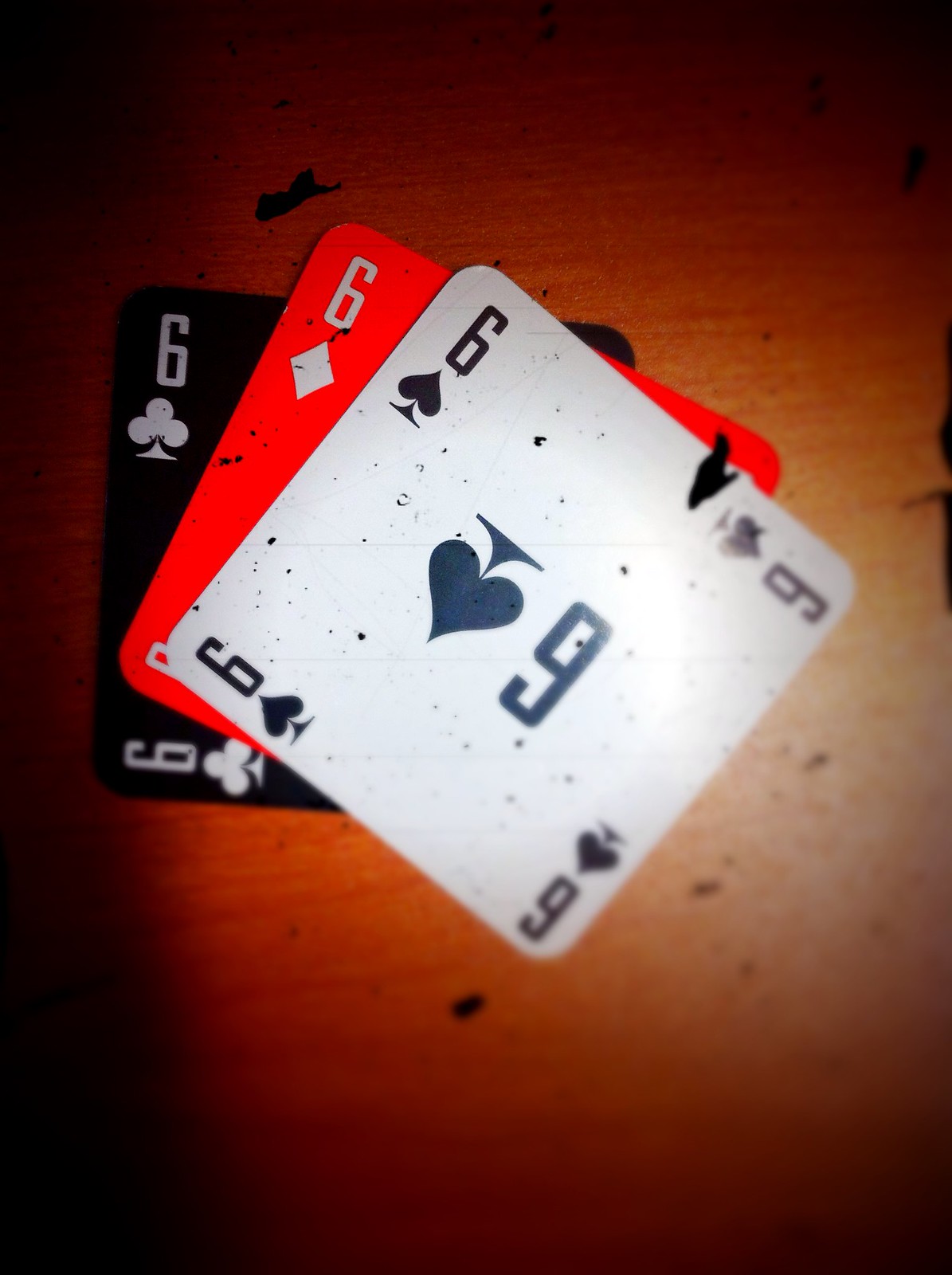A captivating photograph is displayed on a rustic brown wooden table, with the image corners subtly fading to black, creating a vignette effect. Centrally illuminated by a focused light, the table's surface reveals an array of playing cards, scattered and partially obscured by darkness and light. Central to the composition is a fully visible six of clubs card, unmistakable with its crisp white background and black inscriptions. The card prominently features a large number '6' accompanied by the emblematic club symbol both centrally and in the corners. To the left lies the edge of a red six of diamonds card, identifiable by the partial view of its diamond symbol and red hue. Below these, a sliver of another card peeks out, revealing just the corner of a black card adorned with the six of clubs insignia in white. The scene, enriched by subtle details and the interplay of light and shadows, evokes a mysterious and almost cinematic ambiance.